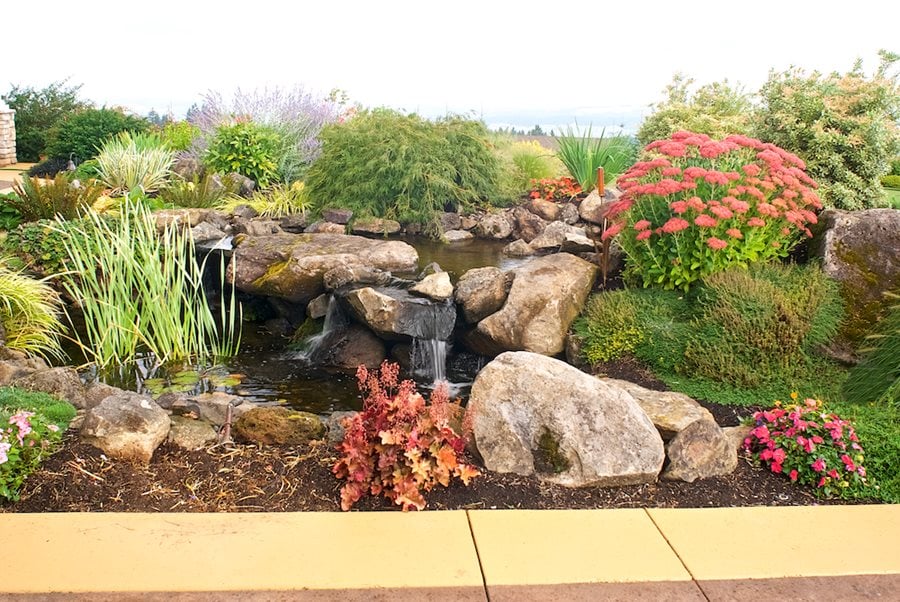This image showcases a meticulously landscaped pond in a suburban setting, framed in a horizontal-rectangular format. In the forefront lies a yellowish sidewalk, leading to a lush garden teeming with diverse plants. Prominent grayish-brown boulders structure the scene, with water trickling down to form a serene waterfall that feeds into the mossy green-brown pond. The pond itself is adorned with lily pads and surrounded by a variety of plants, including tall reeds emerging from the water.

Immediate attention is drawn to the vibrant plant life: an orange plant takes center stage in the front amid two large gray boulders, while a smaller red plant is situated nearby. Above them blooms a striking plant with coral-colored flowers, flanked by abundant grasses and bushes that add layers of greenery. To the right of the waterfall, a large reddish bush displays its red flower tops prominently, accompanied by shorter, pinkish flowers in a nearby flower bed. This well-crafted garden exudes tranquility, blending natural elements with artistic garden design.